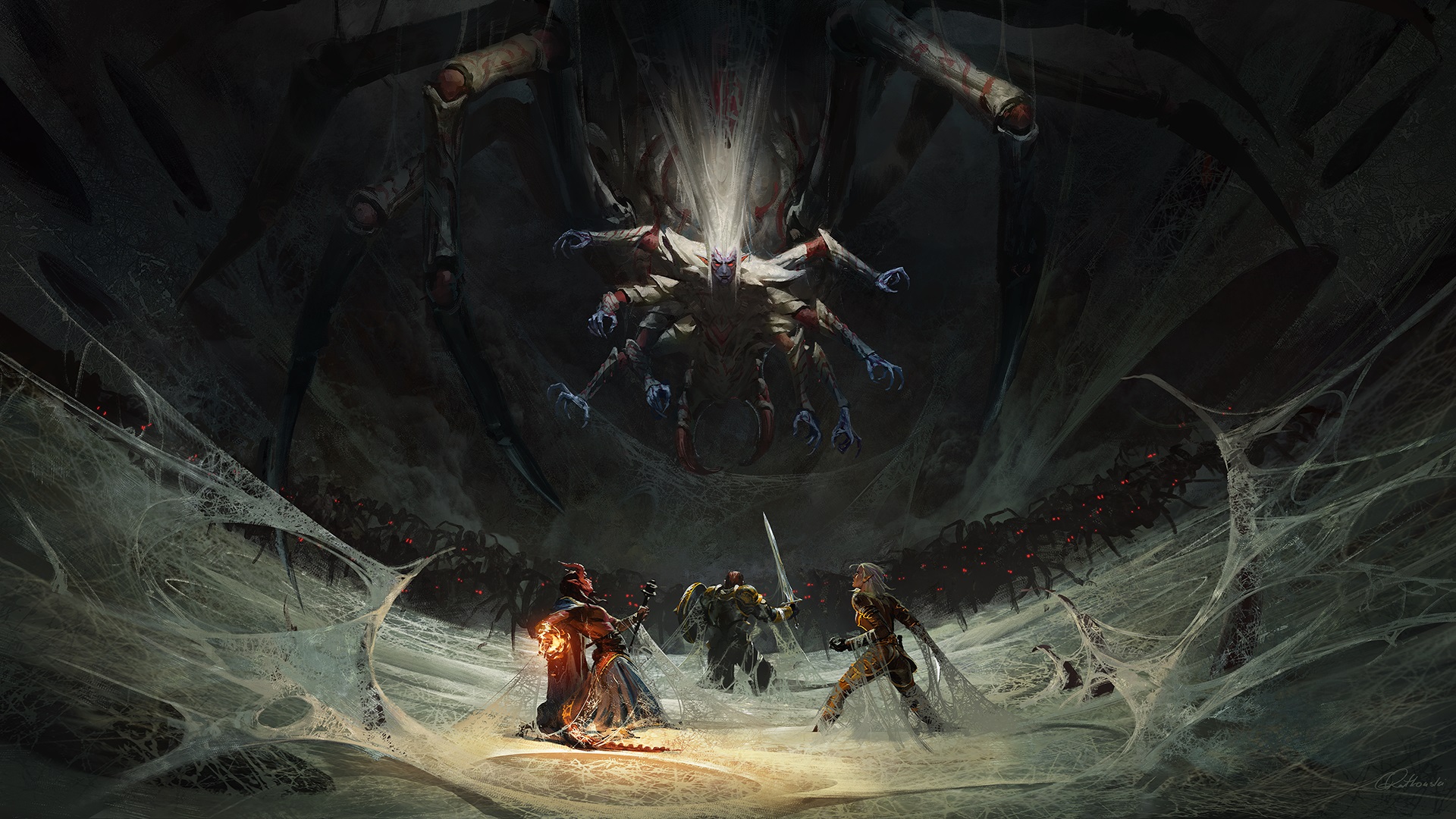In an ornately detailed fantasy illustration, the scene is set inside a giant, monstrous spider’s lair with a dark, cavernous ceiling. The dim environment is eerily illuminated from below, casting light on a terrifying figure that is a hybrid of spider, human, and robot. This creature, itself a grisly spectacle, has a body adorned with red speckles and blue, human-like hands attached to its multiple legs. Surrounding these legs are additional spider limbs, contributing to its monstrous appearance. Suspended in a vast network of cobwebs that envelop the floor, three human figures find themselves ensnared. One man, seemingly their leader, raises a sword defiantly, while the other two struggle within the sticky confines of spider silk. Descending from the darkness above, the intimidating hybrid looms over them. Meanwhile, an oncoming horde of black-bodied spiders with menacing red eyes approaches, heightening the tension of the impending battle. The ornate design suggests elements of science fiction blended with fantasy, as evidenced by the interplay of humanoid and spider-like features within the mysterious lair.